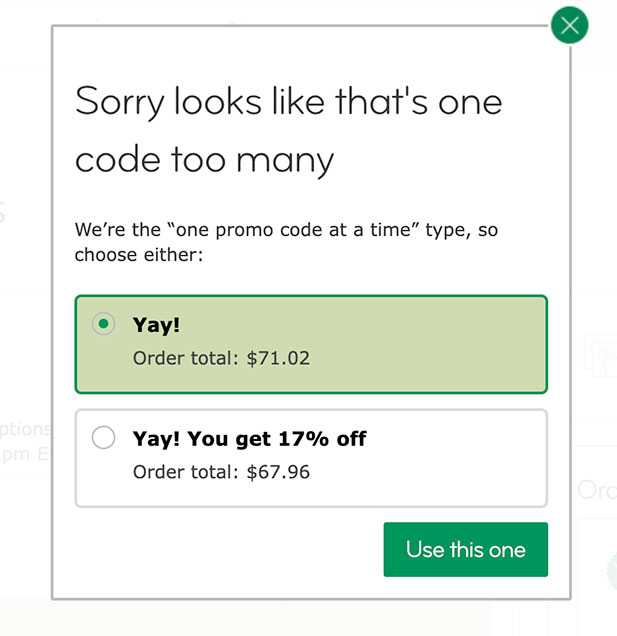In the image, there is a pop-up menu with a black background and a grey outline. In the top right corner of the pop-up, there is a green circular button with a white 'X' inside it, which is used to close the menu. Prominently displayed in the center of the pop-up are the words: "Sorry, looks like there's one code too many." Below this, a message states: "We are the one promo code at a time type, so choose either."

The pop-up presents two promo code options:

1. The first promo code reads "Yay! Order total: $71.02." This option is highlighted with a green outline, and there is a checked checkbox to its left, indicating it is currently selected.
2. The second promo code reads "Yay! You get 17% off, then order total is $67.96." This option is not selected, and its checkbox remains unchecked.

At the bottom right of the pop-up, there is a green button with white text that says "Use this one." This button, colored green, denotes that the currently selected promo code is the first one.

The background of the main page is slightly visible behind the pop-up menu, with some content peeking out from the bottom left corner where the word "Options" is partially revealed.